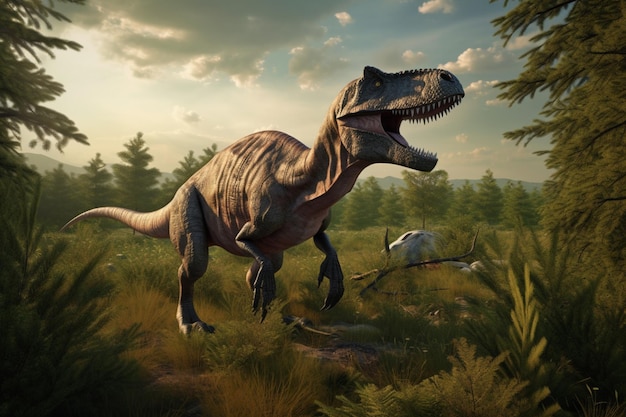This is a digital illustration depicting a T-Rex dinosaur in a lush, forested environment. The large T-Rex, painted in brownish and possibly grayish green or blue hues, stands prominently in the middle of the frame on its two legs with a long, thick tail extended behind. It faces the right side of the image with its mouth wide open, revealing an array of sharp teeth. The dinosaur's small arms hang down as it appears to be in a running stance. The forested background features various pine and fir trees, their green foliage densely packed to the left and right of the T-Rex, framing it naturally. The sky above is a light blue, dotted with gray and white clouds, and it casts a light source from the upper left, creating shadows on the dinosaur. In the distant background, there are rolling hills or mountains, adding depth to the scene. The ground beneath the T-Rex is grassy with some fallen branches and a rock visible next to it, enhancing the wild and rugged terrain.